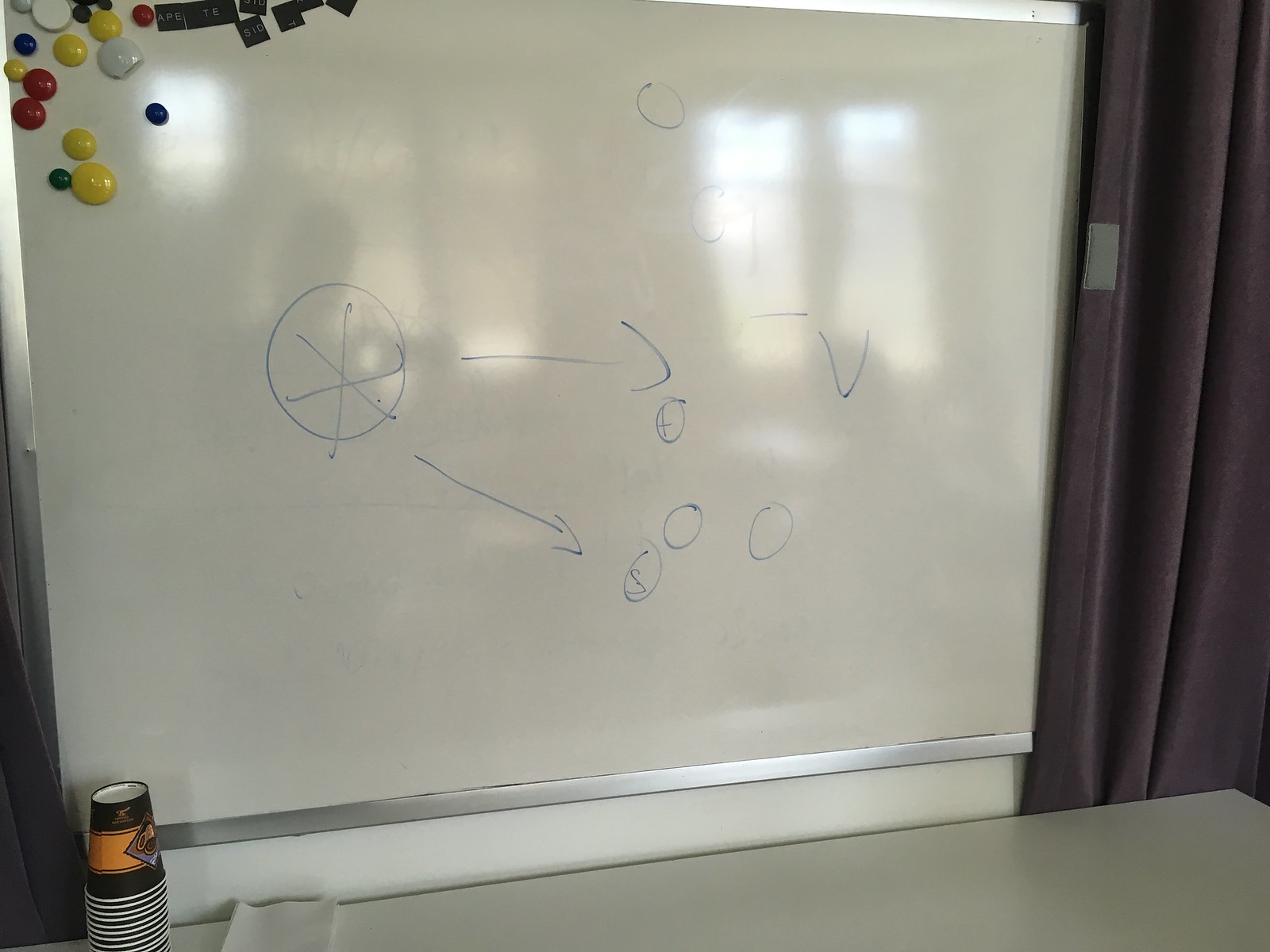A whiteboard, measuring approximately three feet high by four feet wide, forms the central focus of this image. In the upper left-hand corner, a collection of small, circular magnets, comparable in size to M&Ms, is arranged. The magnets are vibrant, featuring colors such as yellow, red, blue, gray, and white.

The whiteboard itself displays minimal markings, all in blue marker. Near the top center, a few circles are drawn. Beneath these circles, the letter "V" is situated, with another circle to its left. This particular circle is unique as it contains a line and a cross through its center, accompanied by an arrow pointing to the right and another angled towards the five o'clock position. Additionally, four more dots are scattered nearby.

A gray curtain hangs to the right of the whiteboard, adding a background element to the scene. Below the board, on a table positioned in the bottom left corner of the image, several paper cups in orange and black hues are placed, contributing a splash of color to the lower part of the frame.